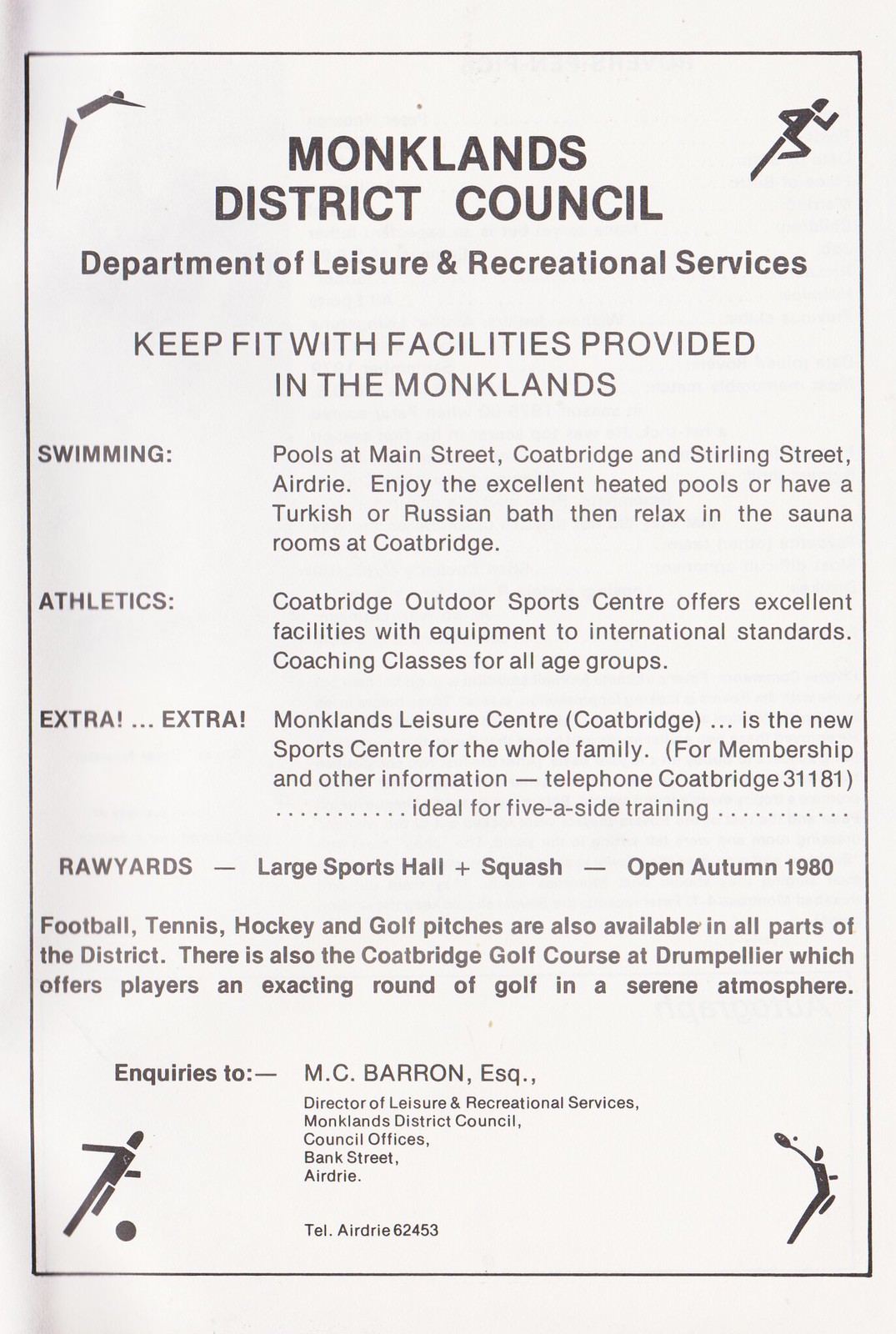The poster features a white background with a small black rectangular border and detailed black text. At the center, in large capital letters, it reads "Monklands District Council," followed by "Department of Leisure and Recreational Services" in smaller text below. The content encourages residents to "Keep fit with facilities provided in the Monklands."

The facilities include swimming pools at Main Street, Coatbridge, and Stirling Street, Airdrie, where visitors can enjoy excellent heated pools, Turkish and Russian baths, and relax in sauna rooms at Coatbridge. For athletic activities, the Coatbridge Outdoor Sports Centre offers excellent facilities with international standard equipment and coaching classes for all age groups.

Highlighted under "extra extra" is the Monklands Leisure Centre in Coatbridge, a new sports center for the whole family, and ideal for five-a-side training. For membership and other information, it provides the phone number Coatbridge 31181. Additionally, Raw Yards Large Sports Hall offers squash and was slated to open in autumn 1980.

Other activities mentioned include football, tennis, hockey, and golf pitches, available throughout various parts of the district. The Coatbridge Golf Course at Drumpellier offers players an exacting round of golf in a serene atmosphere. For inquiries, contact M.C. Barron Esquire, Director of Leisure and Recreational Services, at the Monklands District Council, Council Offices, Bank Street, Airdrie, or by phone at Airdrie 62453.

The poster also features small 2D images in each corner depicting stick figures engaging in different sports: diving or gymnastics in the top left, running in the top right, playing basketball or football in the bottom left, and playing tennis in the bottom right.